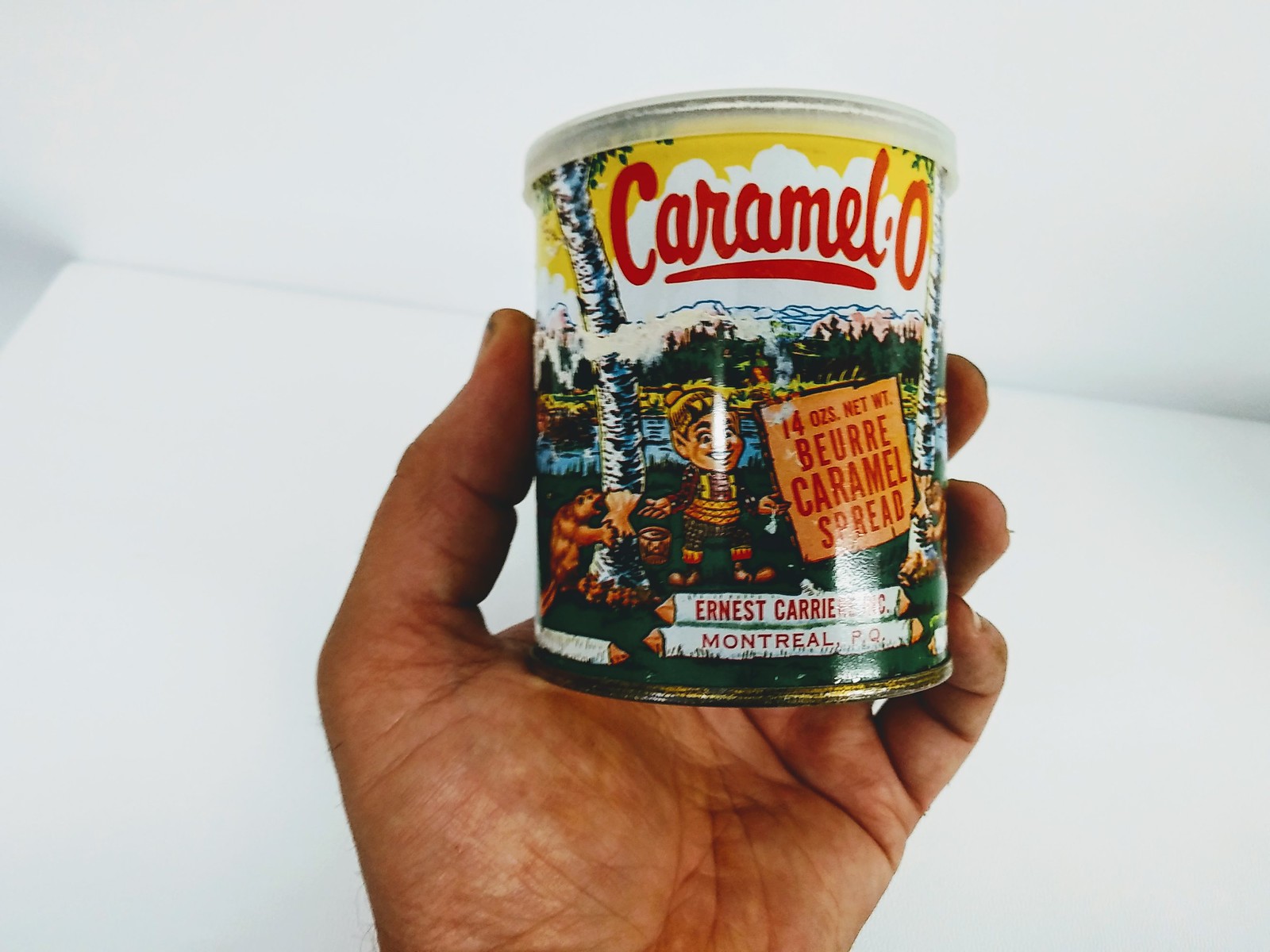The image depicts a tan hand, specifically the palm, holding a colorful can of food with a clear, light white plastic top. The can, designed in a vintage 1950s-40s illustrator style, prominently features a festive label with yellow, white, and red hues. At the top of the label, a yellow sky with a large billowy cloud frames the word "Caramello" written in red cursive. Below the logo, the scene depicts a cartoon boy with blonde hair, light skin, and a slightly deranged smile, dressed in attire reminiscent of lederhosen. He stands next to a wooden sign that indicates "14 ounces net weight" and "Caramel spread." The background displays mountains, a lake, pine trees, and perhaps a beaver or bear to the left, contributing to the busy and visually rich design. Near the bottom, partially obscured, is the text "Ernest Carey's," followed by "Montreal, P-O."